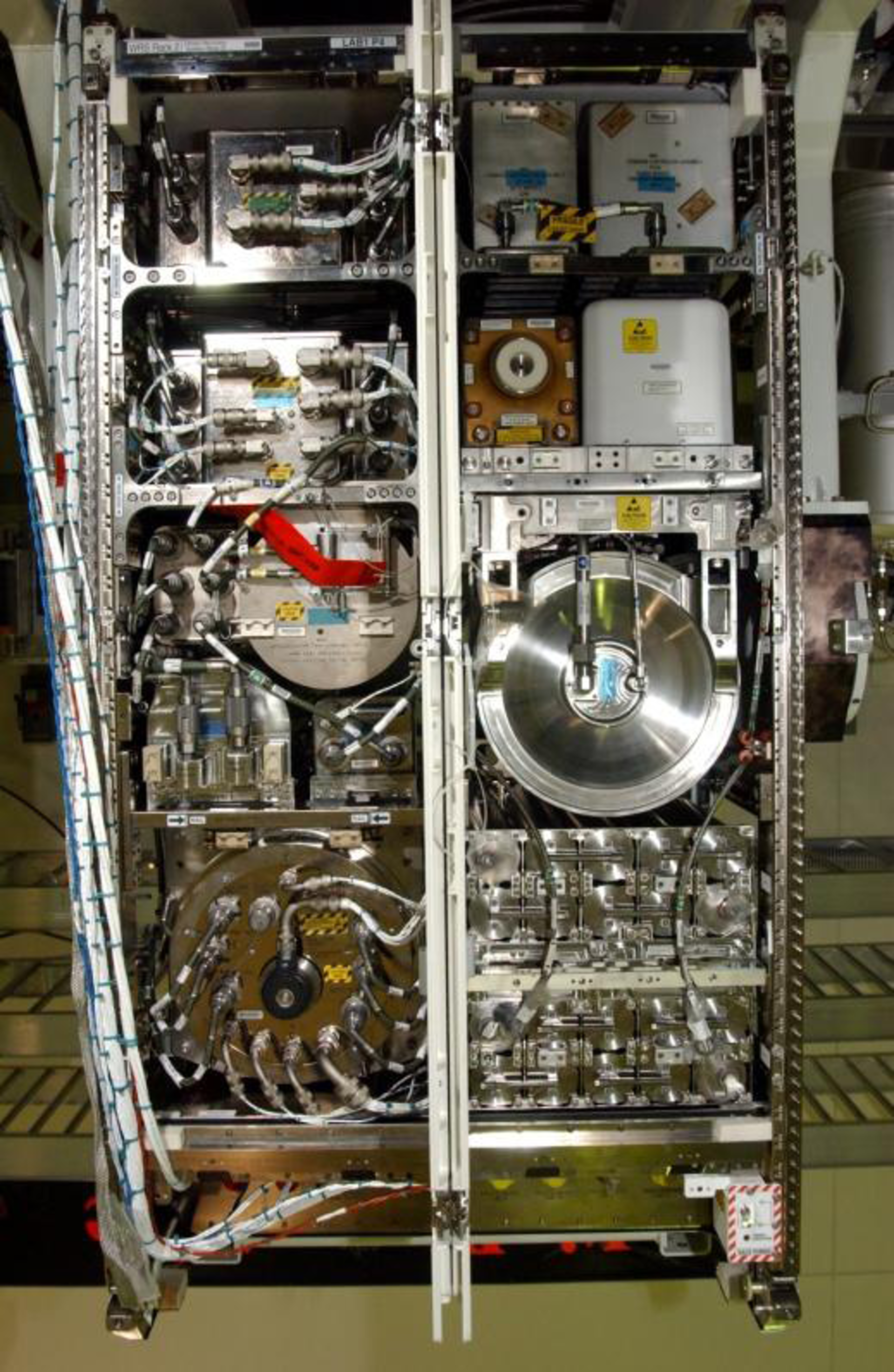This detailed photograph captures an intricately assembled piece of industrial machinery housed in an indoor setting. The focal point is a long, rectangular metallic shelf positioned on the floor, replete with assorted electronic and electrical components. Arranged in numerous sections, the shelf showcases an array of metallic items predominantly in silver hues, complemented by occasional golden components. These elements appear to be interconnected by an extensive network of wires running along the entire structure.

To the top right, a collection of white boxes can be observed, with additional white cylindrical bodies visible behind the shelf, hinting at other equipment within the room. The machinery is set within a steel framing, and two tall, side-by-side racks can be seen, each vertically standing and brimming with components. On the right-hand shelf, lower sections feature large rectangular boxes adorned with shiny silver knobs, while higher sections hold a notable cylindrical drum followed by white boxes connected by piping.

The left-hand shelf mirrors this complexity, presenting a significant silver cylindrical tube at the lower section, detailed with metal pipes extending to various parts. Higher up, additional metal boxes and components are interconnected with an intricate array of metal piping and tubing. Some components are well-polished and reflective, while others, particularly the rectangular boxes, are made of plastic and bear numerous warning labels.

Giving it an almost ethereal quality, the entire assembly appears slightly suspended, suggesting it is delicately poised above the floor, reminiscent of an advanced scientific laboratory setting or a highly specialized industrial station. Each part, meticulously connected by numerous wires and valves, underscores the complexity and technical sophistication of the machinery.